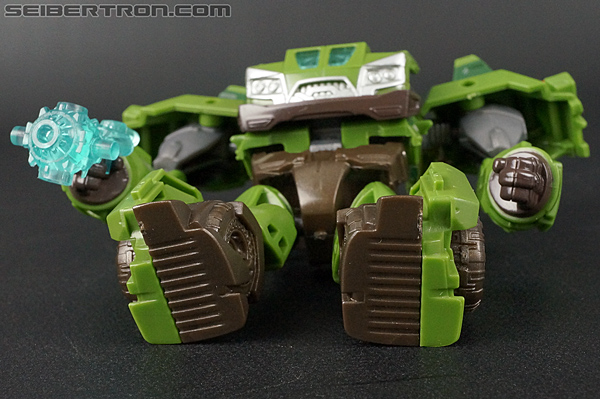The image shows a detailed advertisement for a children's toy prominently featuring a green and brown robot resembling a Transformers character, as indicated by the brand "Cybertron.com" in the upper left corner. The robot is reclined backwards on a black surface, showcasing its large, broad shoulders and intricate parts designed to fit together for transformation. Its face, modeled to look like the front of a truck, has blue eyes and silver details, with silver also visible in the underarm areas due to its tilted position. The robot's hands, one of which is gripping a teal-colored weapon, and feet, which are two-toned in green and brown, are intricately detailed. Tires are attached to the sides of its feet, adding to the realistic transformation elements. The background is a subtle gray with darker gray lettering for the website, making it slightly challenging to read but emphasizing the figure of the robot toy with its vibrant colors and detailed features.